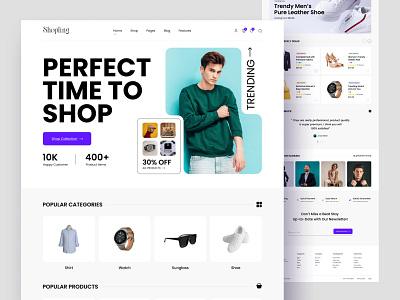The image appears to be an online advertisement, possibly from a webpage, promoting the perfect time to shop with the platform "Shopify" prominently mentioned at the top. It features navigation links in small boxes with black writing that suggest additional pages. Beneath the headline "perfect time to shop," there is a prominent purple button with unreadable text, followed by metrics indicating "10k" in one section and "400 plus" in another, although their exact meanings are unclear.

The right side of the image showcases a young man with short dark brown hair, light-colored skin, wearing a green sweater and light-colored pants, pulling up one of his sweater sleeves. The background behind him is teal. Adjacent to him is an upward-pointing arrow with the word "trending," suggesting the popularity of his outfit.

To the left, there's a section with four small product images labeled "30% off". Below him, another section titled "popular categories" displays a shirt, a watch, a pair of sunglasses, and a white pair of shoes, each with descriptive labels.

Additionally, there is mention of "popular products," indicating further items below, which are not visible in the cropped section of the image. The combination of stylish presentation and detailed categorization suggests a well-organized shopping platform with significant user engagement.